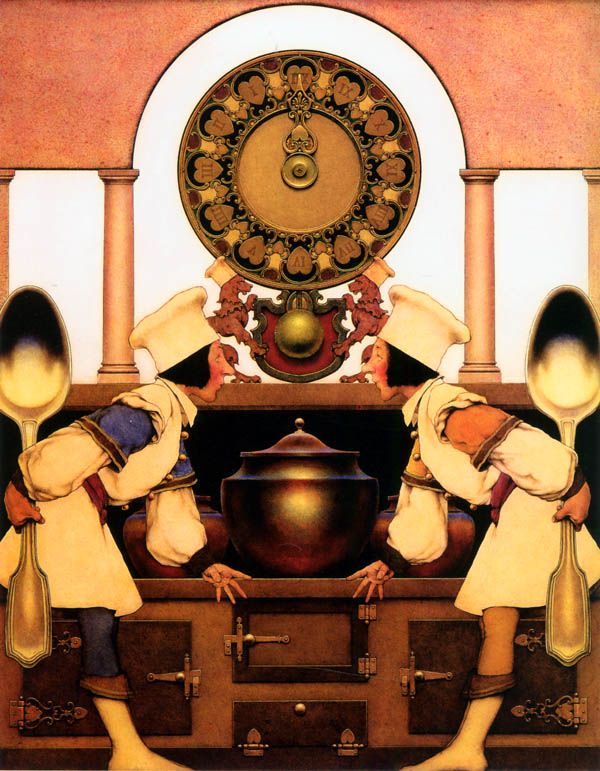The image features a vivid and colorful painting of two identical chefs in a symmetrical arrangement. Each chef is leaning towards the other, their rosy-cheeked faces framed by black, straight hair that falls just below ear-length. Both wear traditional white chef's hats and outfits, but with a distinguishing twist: the chef on the left sports blue sleeves and matching blue pants, while the chef on the right displays orange sleeves with corresponding orange pants. Each chef wields a giant, silver spoon behind their back—one in their left hand, the other in the right—creating a mirrored effect.

Between them, a large black pot with a lid takes center stage, possibly set on a big stove. The chefs’ inside hands rest on or near some brown cabinetry that features an array of locks and hinges. Above this scene, an ornate, circular antique oriental clock acts as a backdrop. At the base of this clock, two rock-like figures of dogs, each donning a chef's hat, seem to uphold the clock. The intricate design and vivid colors add a fantastical element to this already whimsical depiction of chefs in an almost surreal kitchen setting.